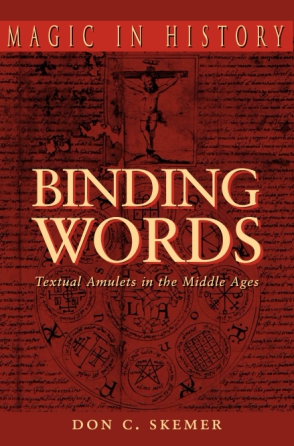The book cover of "Binding Words" features a dark red background adorned with an intricate tapestry of imagery and text. The title, "Binding Words," is prominently displayed in the center in a yellow-orange color with a red drop shadow. Above it, in the same striking yellow-orange hue, the subtitle "Textual Amulets in the Middle Ages" is written. At the very top of the cover, within a red rectangle, the words "Magic and History" appear in the same yellow-orange color. The author’s name, Don C. Skemer, is positioned at the bottom, also in yellow-orange text.

Dominating the background, a depiction of Jesus on the cross occupies the top middle section, surrounded by various symbols and circles. A larger circle is centrally placed with eight smaller ones encircling it, each containing distinct, though somewhat indiscernible, symbols and grids. Some background text appears slightly burnt, particularly in the upper left section, adding a historical and mystical aura to the cover. The overall colors of the cover are red, black, cream, and yellow-orange, with the text exclusively in uppercase lettering.